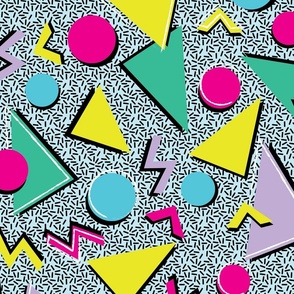This image portrays a vividly abstract pattern reminiscent of 1980s pop illustrations, ideally suited for wrapping paper or a scrapbook background. The artwork is housed in a perfectly square frame with a pale aqua background, adorned with a myriad of small black lines that scatter in all directions, creating a dynamic sense of movement. Overlaying this backdrop are various geometric shapes in bright, eye-catching colors. The most prominent shapes include large and medium triangles in shades of yellow, pale green, and lavender; circles in hot pink and sky blue of varying sizes; and zigzag lines and chevron-like V-shapes in yellow, hot pink, and yellow zigzag. Some of these elements are outlined in black, enhancing their bold presence. In total, approximately 20 distinct shapes are arranged purposefully within the image, including three blue circles, three and a half yellow triangles, two and a half green triangles, five hot pink circles, and three yellow V-shapes, among others. The overall composition evokes a playful, energetic aesthetic characteristic of its era.